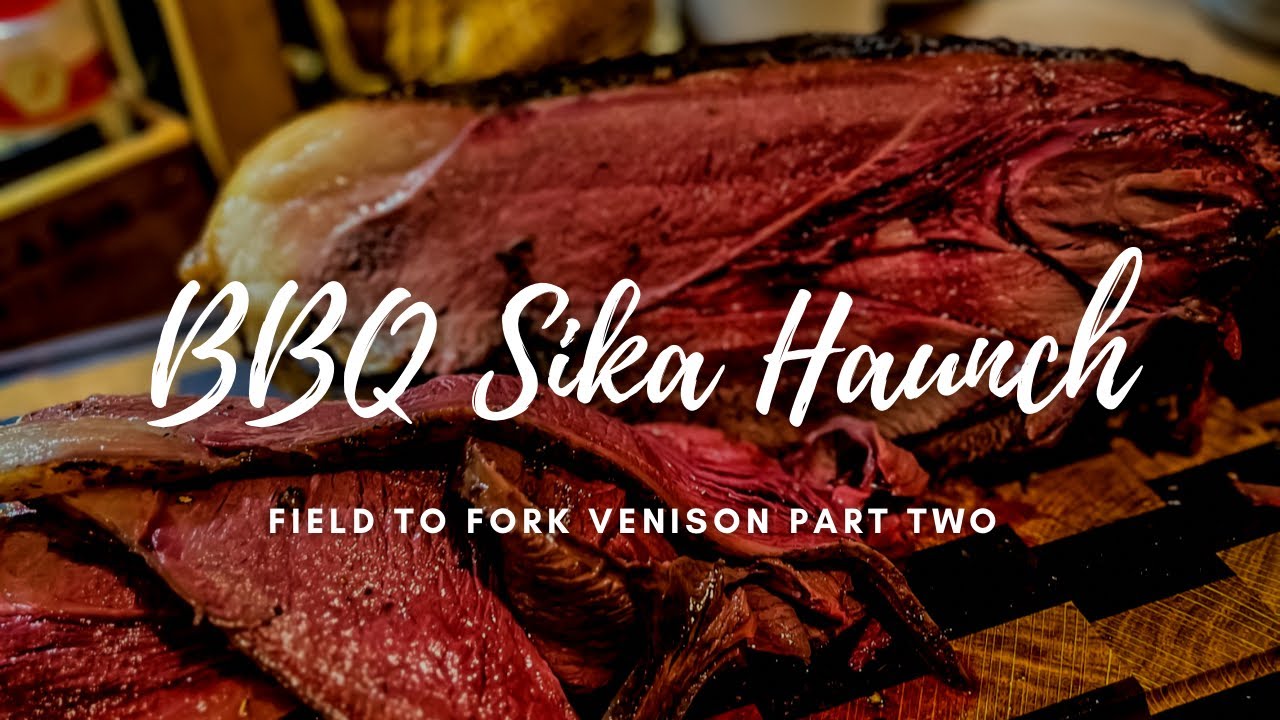The image is a close-up photograph showcasing a piece of rare, red venison meat on a black-and-white checkered cutting board. The meat, advertising "BBQ Sika Haunch Field to Fork Venison Part 2", is prominently displayed with a significant chunk of fat on the left side. Slices of the venison are falling naturally in front of the main piece, emphasizing its raw and bloody appearance. The background features indistinct, blurry objects in beige and dark colors, possibly a cabinet, adding to the rustic and artisanal feel of the presentation. The caption and setting position it as both food art and an advertisement for venison.